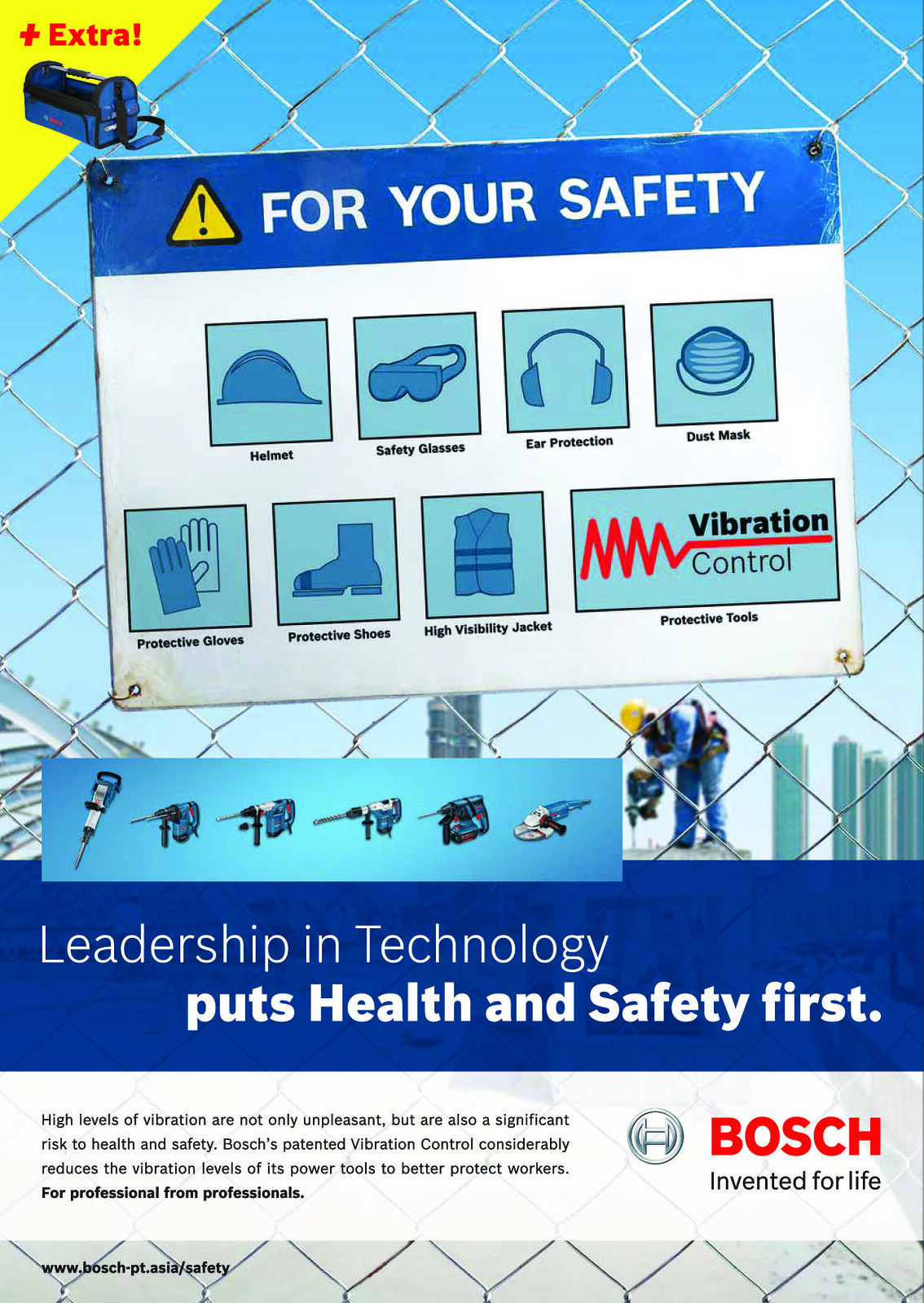The image presents an advertisement poster set against a background resembling a chain-link fence, with a construction worker donning a yellow hard hat visible behind the fence. The poster dominates the entirety of the image and is geared towards promoting workplace safety, particularly highlighting Bosch's commitment to reducing tool vibration for worker health and safety.

At the top of the poster, the phrase "Plus Extra" is inscribed. Adjacent to this, a yellow mailbox icon adds to the array of visuals. Beneath this header, a prominent section labeled "For Your Safety" is encased in a blue bar with an accompanying hazard triangle containing an exclamation mark.

This section features illustrations of various safety gear, each in its own square box: a helmet, safety glasses, ear protection, and a dust mask. Below these are four larger boxes outlining additional safety equipment: protective gloves, protective shoes, a high-visibility jacket, and vibration control tools. A distinctive red, seismograph-like graphic with the label "Vibration Control" draws attention to Bosch’s patented vibration control technology.

The lower part of the poster showcases six Bosch power tools followed by a blue bar with white text reading, "Leadership in technology puts health and safety first." Below this is a gray rectangle containing detailed information about the health risks associated with high tool vibration and Bosch's efforts to mitigate these risks through their patented technology. The paragraph ends with the tagline, "For professionals from professionals."

To the right of this text block, the Bosch logo is prominently displayed, with "Bosch" in large red letters and the motto "Invented for life" in smaller black text beneath it. Finally, the website address "www.bosch-pt-asia-safety" is listed at the very bottom. The overall color scheme of the poster incorporates shades of gray, black, white, red, dark blue, light blue, and yellow, reinforcing its visual impact and emphasis on safety.